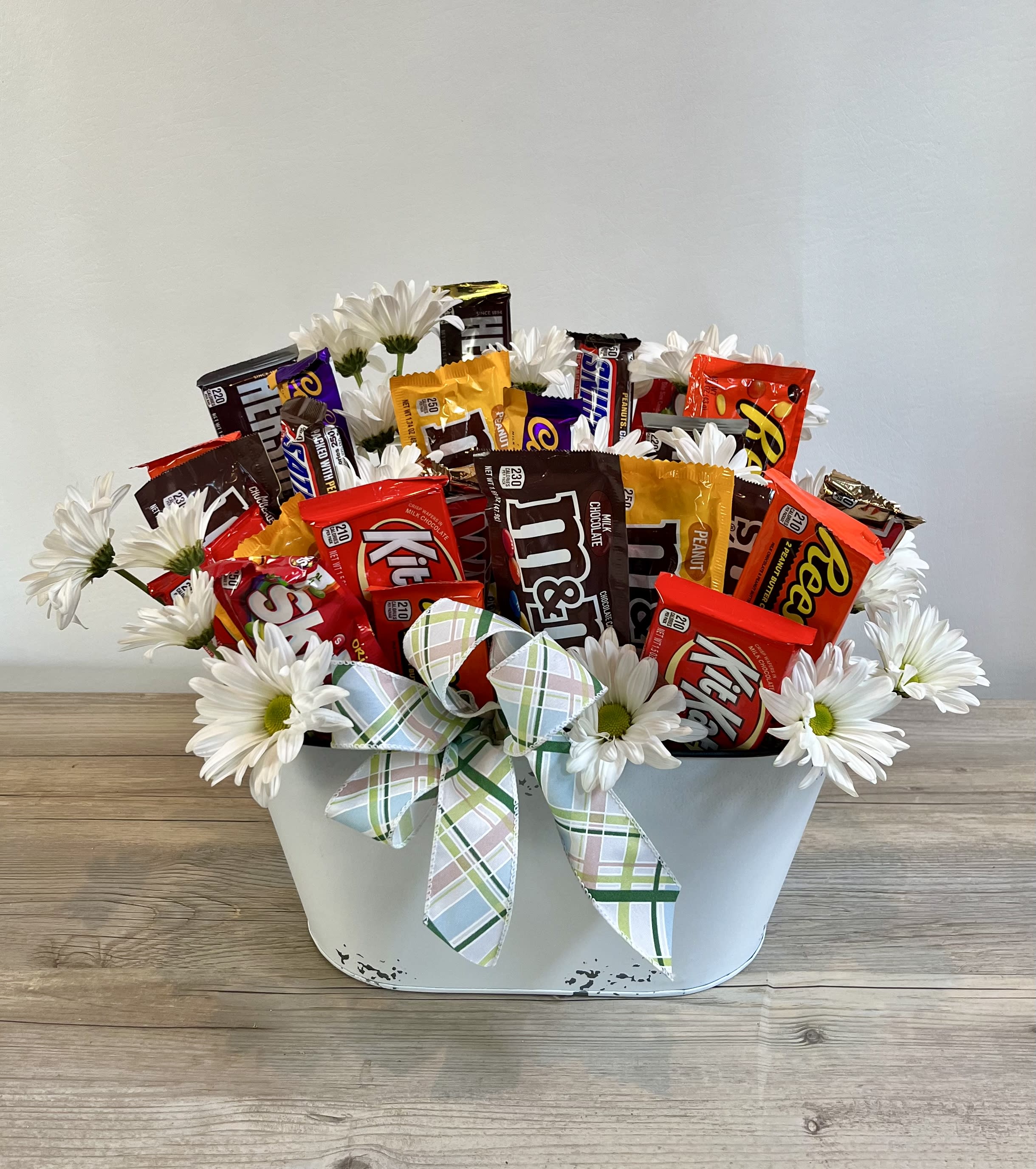The image depicts a rustic, white, metal planter basket situated on a light wooden surface. The planter, with its chipping paint revealing a silver metal underneath and gray specks, exudes a vintage charm. Adorning the basket is a festive, spring-colored plaid ribbon featuring hues of pink, light green, dark green, white, and light blue. Nestled within the planter and peeking out among the contents are small white daisies, adding a delicate touch of nature. The centerpiece of the arrangement is an assortment of candy bars, meticulously arranged to resemble a bouquet. The selection includes Kit Kats, Skittles, plain and peanut M&M's, Reese's Pieces, Snickers, Hershey bars, Twix, Carmelo bars, and possibly a Mars bar. This delightful candy bouquet, set against a gray wall, makes for a charming and cheerful gift.